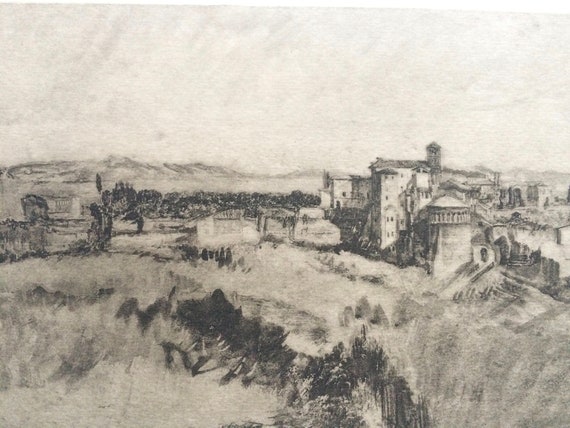The image is a monochrome drawing, likely executed in pencil or charcoal, depicting a serene countryside scene with a historical or old-town European feel. The setting is outdoors, and the sky occupies the top portion of the square, borderless image. In the distance on the left side, rolling hills and small trees create a gentle backdrop, while barely visible, light-gray mountains faintly outline the horizon.

In the foreground, detailed charcoal strokes represent grass and shrubs, lending a textured realism to the scenery. The midsection of the image showcases a town with various buildings. To the center right, there are several multi-story structures, including a distinctive building with a rotunda, reminiscent of an old grain silo. Another prominent building features multiple windows and a notable roof, hinting at its historical architecture. Some buildings are blurred, adding depth and a touch of mystery to the scene.

Overall, the detailed and soft rendering of the drawing imbues it with a tranquil yet timeless quality, portraying a countryside townscape viewed from an elevated position.